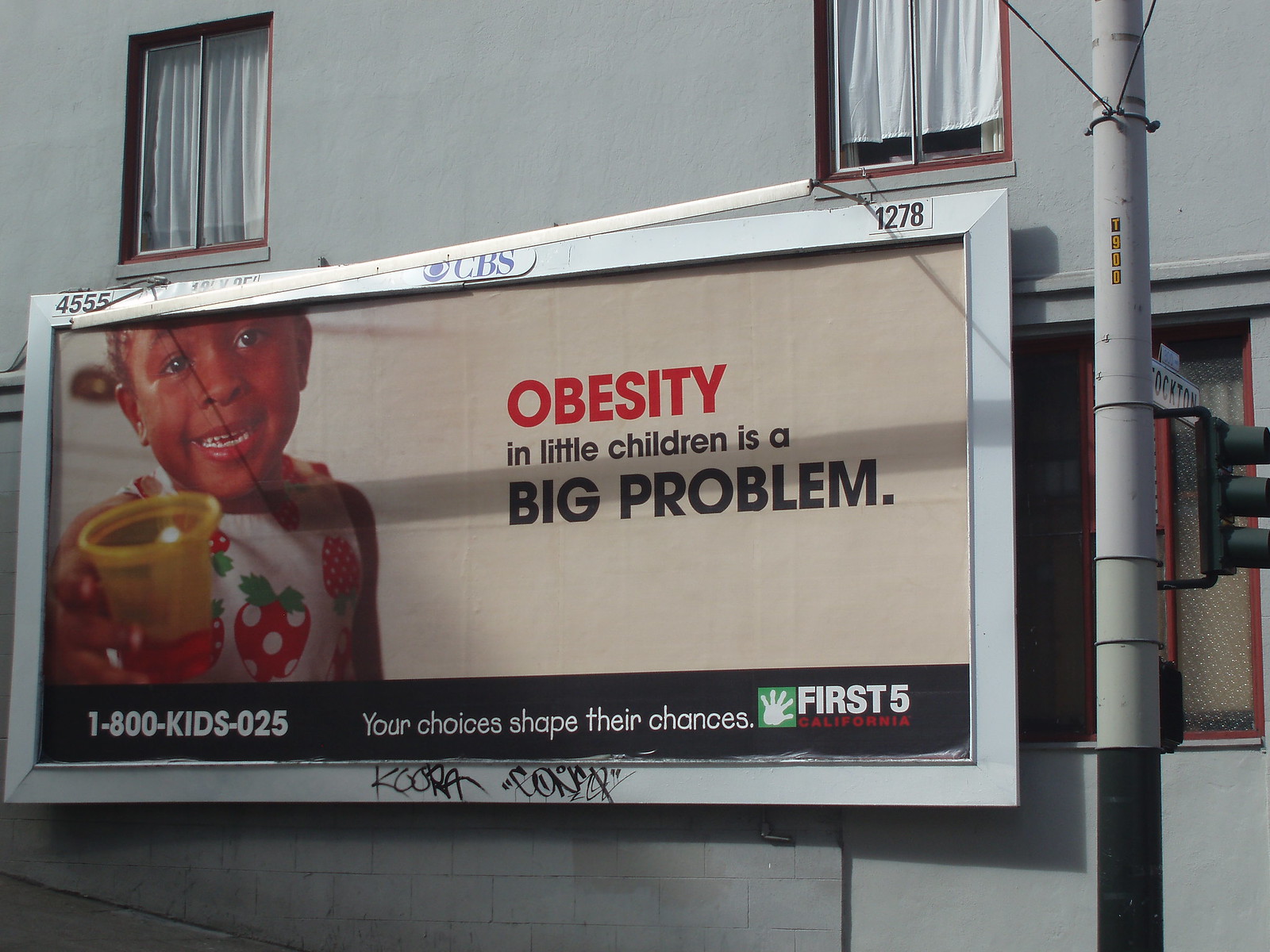The image depicts a large rectangular billboard attached to the side of a concrete building, possibly an apartment complex. The billboard is framed in metal, with "4555" in numbered stickers on the top left corner and "1278" on the top right. The CBS logo is centered at the top of the billboard. The main visual shows an African-American child wearing a white shirt adorned with animated strawberries, holding up a yellow plastic cup filled with juice. The prominent text on the billboard reads, "Obesity in little children is a big problem," with "obesity" in red and the rest in black lettering. At the bottom of the billboard, a black banner displays the message "Your choices shape their chances," along with the phone number "1-800-KIDS-025," and the "First 5 California" logo on a green background with a white hand stamp. The billboard's frame and the concrete wall beneath it have visible graffiti. To the right of the billboard, a gray and black traffic signal pole is partially visible, with a black traffic light and an out-of-focus road sign. The background showcases the light gray concrete blocks of the building and two windows at the top of the image.